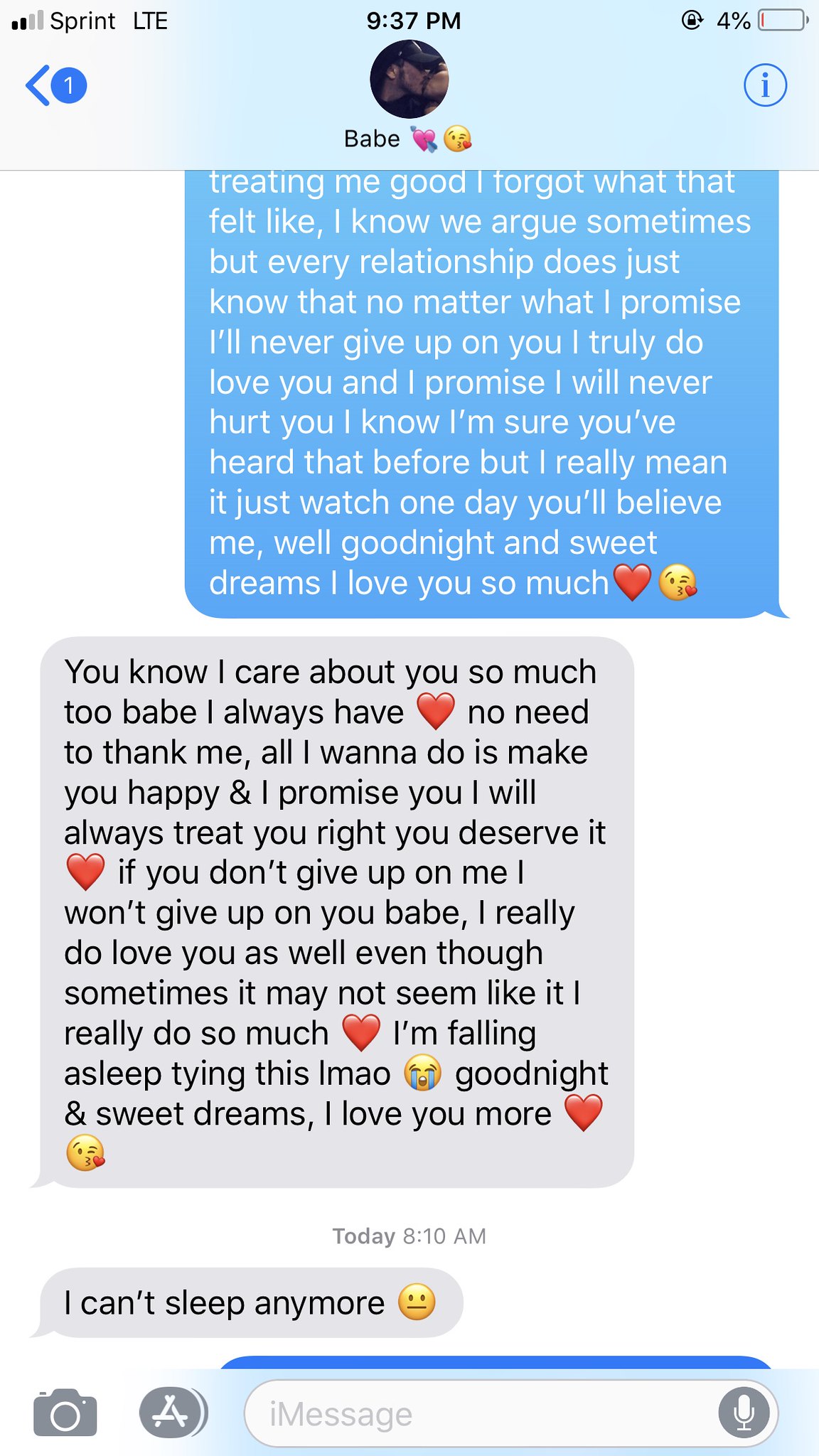A detailed screenshot of a text message exchange between two people labeled as "Babe ❤" in a chat interface on a Sprint LTE phone with 4% battery life (indicated in red) at 9:37 PM. The conversation involves an affectionate dialogue with emotional expressions:

In a blue bubble, "Babe ❤" sends:
"Treating me good, I forgot what that felt like. I know we argue sometimes, but every relationship does. Just know that no matter what, I promise I'll never give up on you. I truly do love you and promise I will never hurt you. I know, I'm sure you've heard that before, but I really mean it. Just watch, one day you'll believe me. Well, goodnight and sweet dreams. I love you so much. 😘"

The reply, in a gray bubble, states:
"You know I care about you so much too, Babe ❤. I always have. No need to thank me. All I want to do is make you happy, and I promise you I will always treat you right. You deserve it. If you don't give up on me, I won't give up on you, Babe ❤. I really do love you as well, even though sometimes it may not seem like it, I really do so much ❤. I'm falling asleep tying this LMAO 😂. Goodnight and sweet dreams. I love you more 😘."

Following this, a separate gray bubble states: 
"I can't sleep anymore 😐" at 8:10 AM.

The interface displays typical text message colors with white, gray, and blue elements, an area to input messages, a microphone icon, and an information circle next to the contact's name. The background is white, depicting a standard chat application layout.